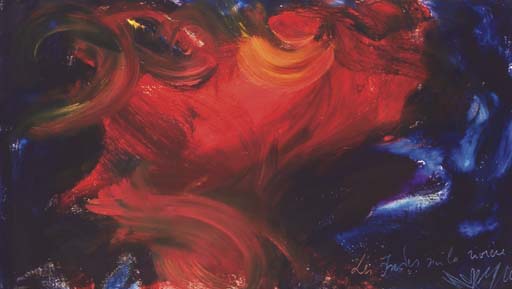This abstract painting features a dynamic composition dominated by intense colors and swirling forms. The centerpiece is a vibrant, fiery cloud-like swirl of red, orange, and yellow hues that rises and spreads across the majority of the painting, resembling a forceful wave or storm. Surrounding this energetic burst, the background is primarily dark, with deep navy blue and black tones on both the left and right sides, accented by hints of purple. Subtle glimmers of white light highlight some of the blue sections, adding depth and contrast. Although there's an artist's signature in cursive at the bottom right corner, it is small and difficult to decipher. Overall, the piece exudes a sense of movement and intensity, typical of abstract art, allowing viewers to interpret the imagery in their own way.